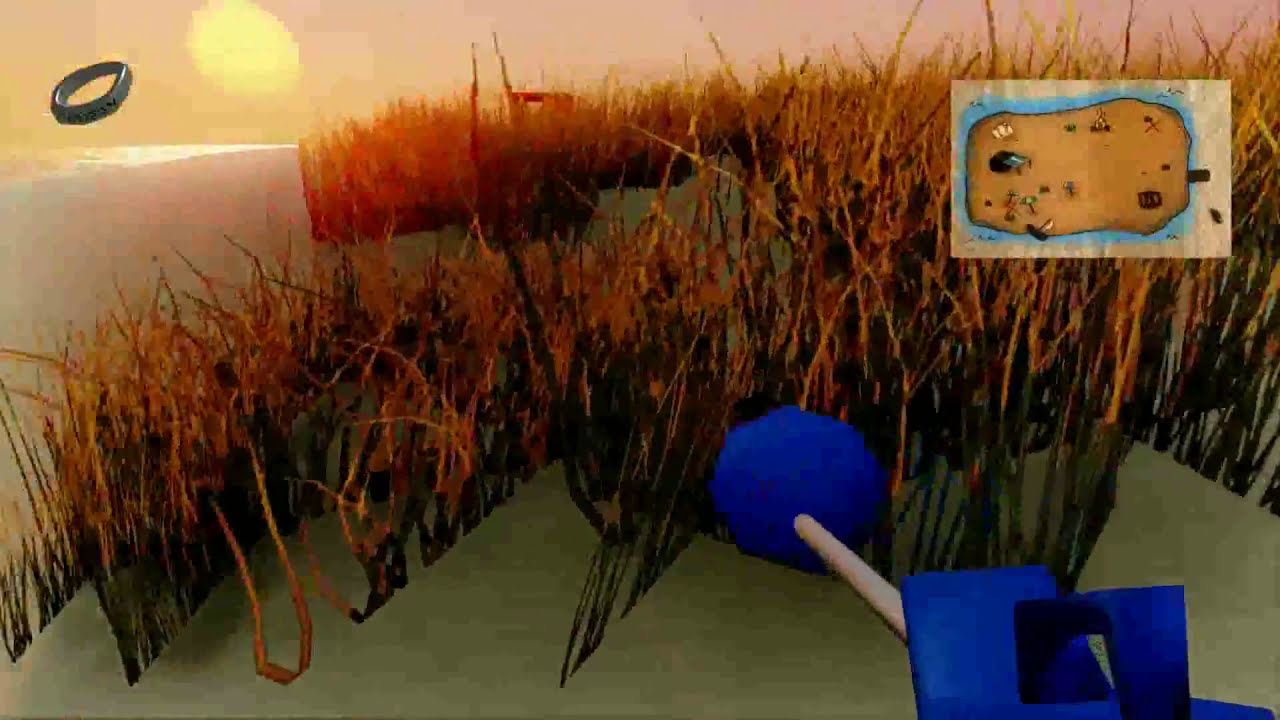This image captures a scene from a 3D video game with rudimentary, blocky graphics in a first-person perspective. In the foreground, there are tall plants resembling reeds or grasses you'd typically find near a pond, but they are withered and lack green leaves, suggesting an autumn or barren environment. This vegetation extends towards the background, where the earthy, dark green terrain is partially visible. In the distance, the sky is illuminated by a sun positioned low on the horizon, indicating dawn or dusk.

In the top right corner of the image, a mini-map displays the current outlying area of the game world, possibly showing various icons for navigation. A ring icon is located in the top left corner, possibly indicating an item of interest, such as a quest objective or discovered object.

Dominating the lower right corner is a blue-colored object that appears to be some kind of detector or tool, potentially akin to a metal detector, characterized by a blue body with a silver shaft and a circular component at the end. This tool is pointed towards the ground amidst the tall plants, reinforcing the notion that the character might be searching for something buried or hidden in this grassy, semi-blocky landscape.